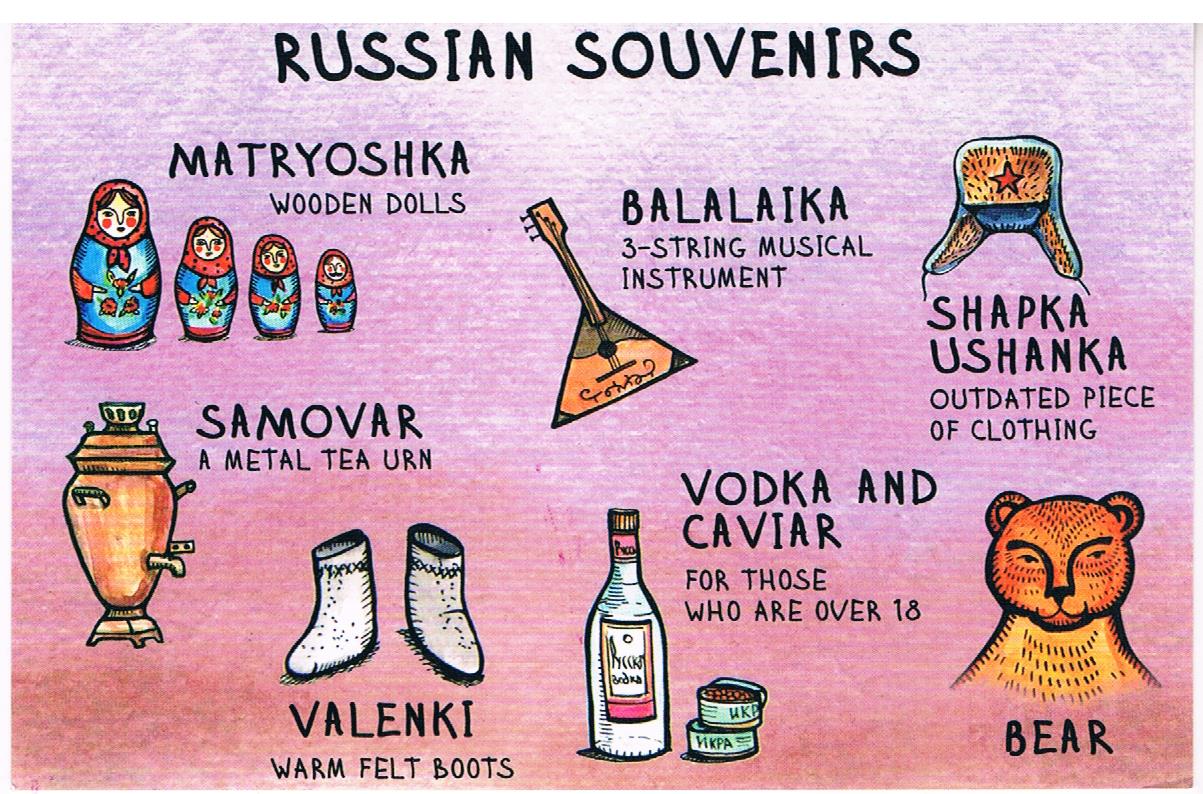The image features a soft, gradient background in shades of purple, white, pink, and reddish tones, creating a smooth visual effect. At the top of the image, the phrase "Russian Souvenirs" is prominently displayed in black letters. Below this title, the text "Matryoshka Wooden Dolls" is written, accompanied by a detailed illustration of four Matryoshka dolls in ascending size order. Each doll has a black body, a red scarf, and rosy cheeks.

Next to the dolls, there is an illustration of a balalaika, a traditional three-string musical instrument. Following this, there is a depiction of a shabka ushanka, a classic Russian fur hat, described as an outdated piece of clothing. Below the hat, the image features a samovar, a tall brown metal tea urn commonly used in Russia.

Further down, the image shows a pair of white valenki, traditional warm felt boots. Accompanying these items, there is a white bottle of vodka and several cans of caviar, indicating these are for individuals over the age of 18. Finally, the illustration includes a detailed drawing of a bear, highlighting another iconic part of Russian culture.